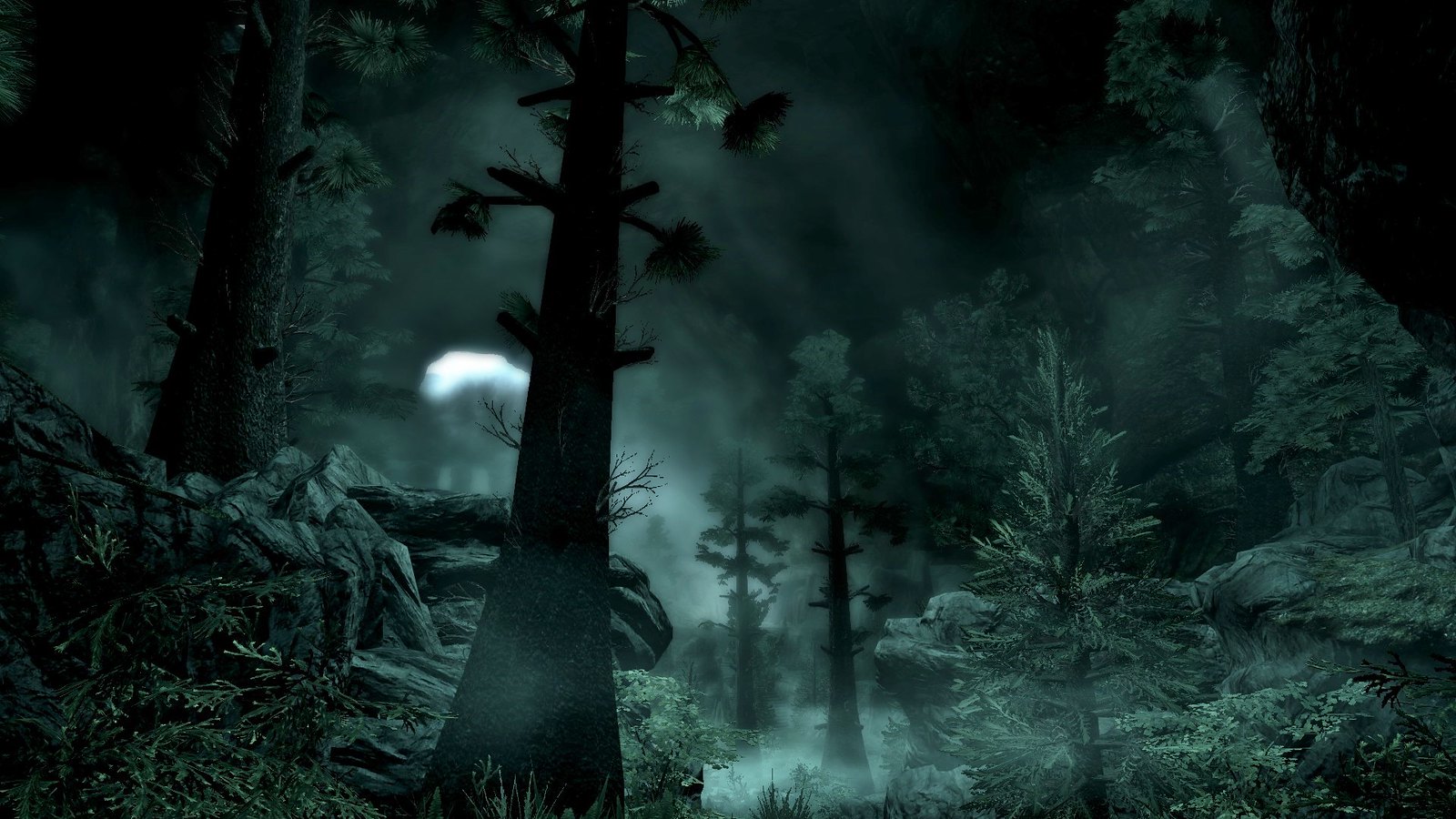This detailed nighttime woodland scene, possibly an intricate painting or a 3D rendering, captures the haunting tranquility of a forest under the moonlight. Dominated by deep, dark hues of green, gray, and black, the scene features two prominent tree trunks on the left, their branches reaching upwards amidst various other trees and bushes. The moonlight, filtering through clouds, casts an illuminating yet shadowy effect on the landscape, highlighting a couple of central trees and creating a mystical, eerie ambiance. On the right, a large rock supports one of the tall trees, with another tall tree behind it, while another rock and several trees populate the left side. Sparse-leaved tall trees contrast with shorter, denser foliage, and a small patch of light penetrates the darkness on the right, adding a touch of ethereal light to the otherwise blurred background. The scene is devoid of any human or animal presence, emphasizing the serene isolation of the nighttime forest.